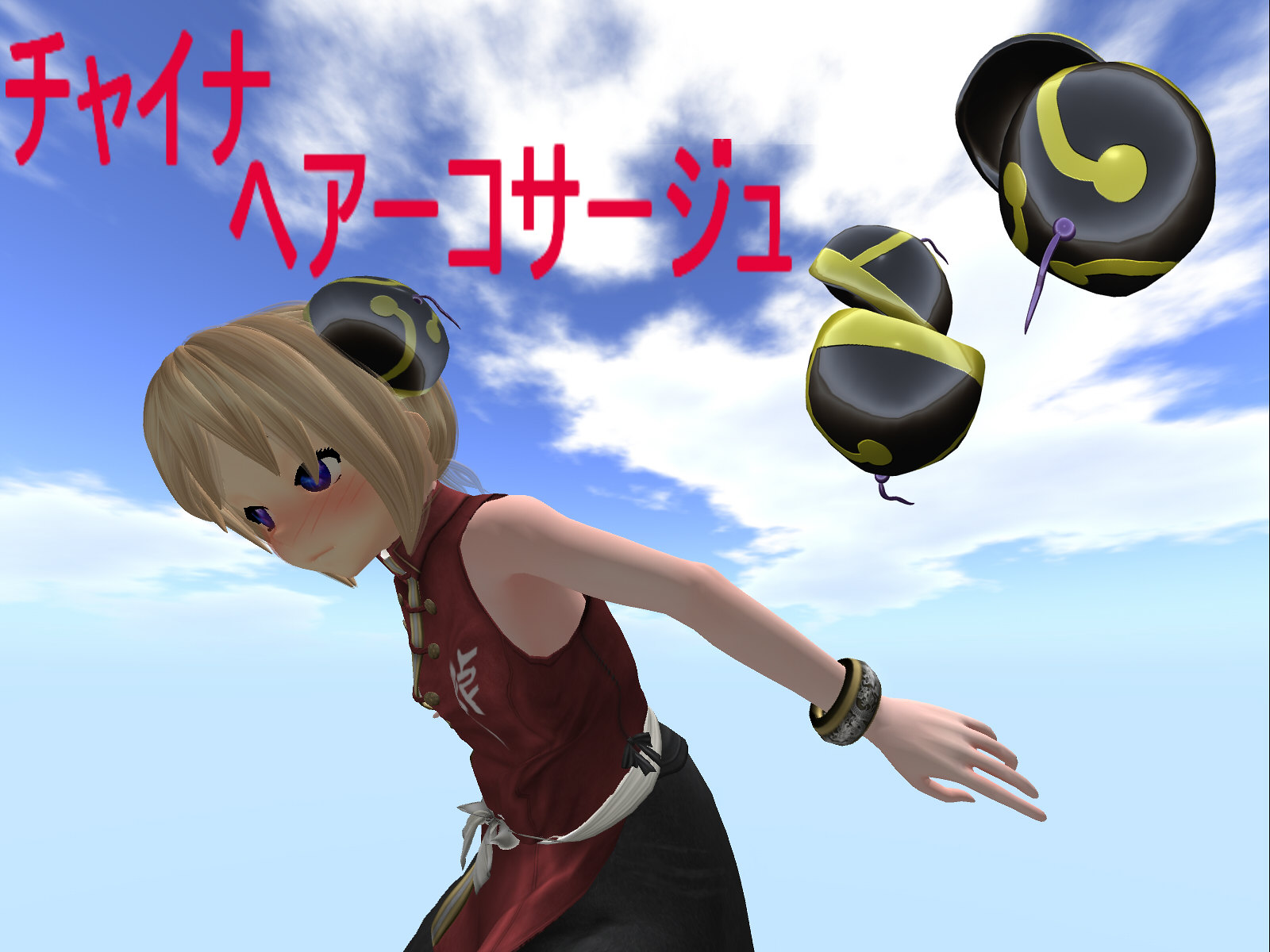The image depicts a scene with a partly cloudy blue sky adorned with wispy white clouds and a lighter blue hue towards the bottom half. In the upper left corner, there's red text written in what appears to be Japanese. Floating in the upper right corner are several round, black and yellow objects that resemble dragon balls or hats. The focus of the image is a female anime character with blonde hair and bright blue eyes. She has a delicate, blushy pink face and is adorned in a scarlet, sleeveless outfit that resembles a vest and skirt, complete with bronze-colored buttons. Tied around her waist is a white linen belt fashioned into a bow. On her raised arm, she wears a large, ornate green and gold bracelet. Additionally, she has a small black hat on her head, mirroring the floating items around her.